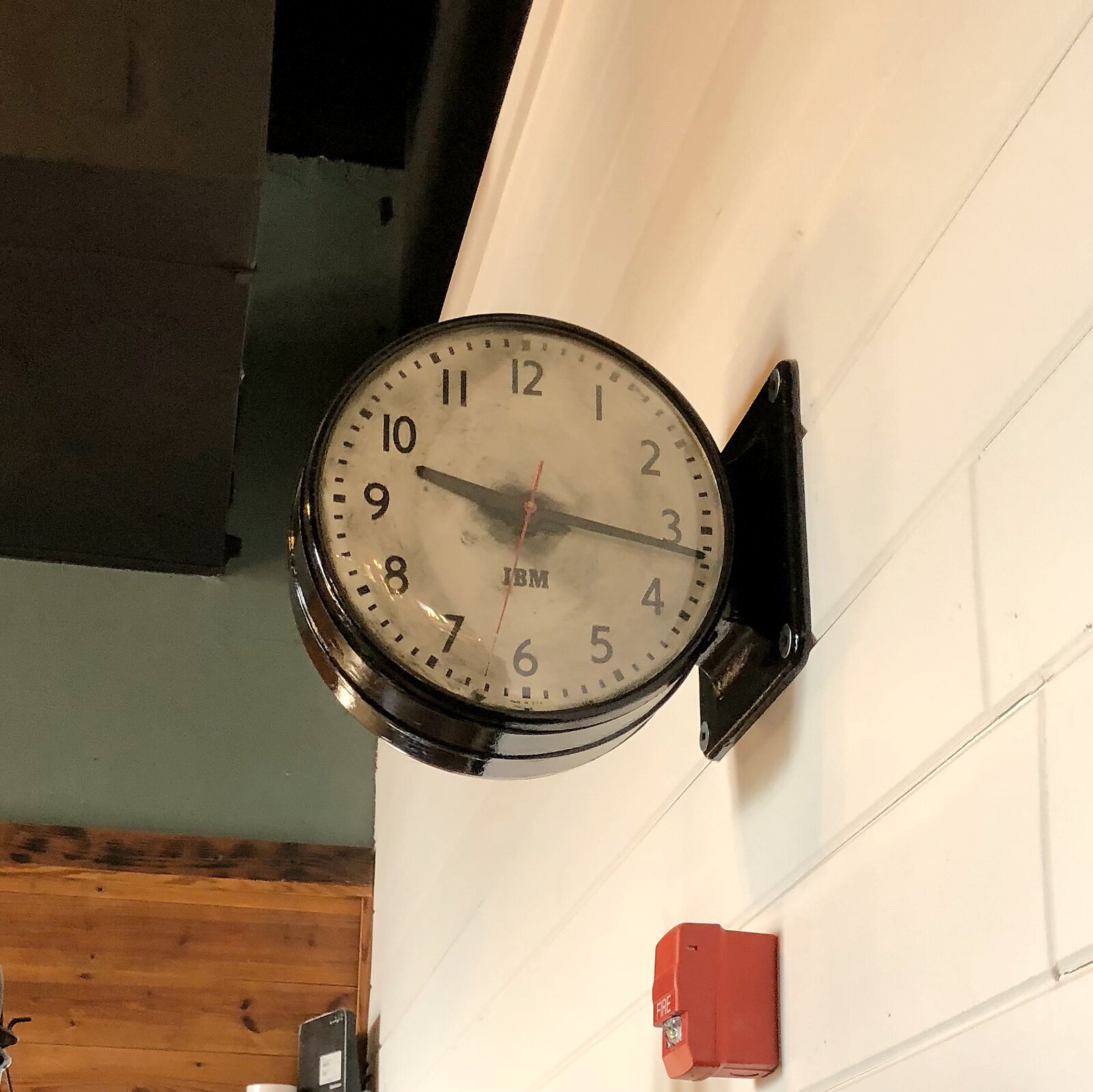The image depicts a photograph of a traditional school clock mounted on a white cinder block wall. The clock is circular, with a black frame and a white dial featuring black numerals from 1 to 12. The hour hand points slightly past the 9, and the minute hand is just past the 3, indicating the time is approximately 9:17. Positioned just below the clock's center is the black text "IBM." 

The clock is affixed to the wall with a black mounting base. Below the clock, there is a prominent red fire alarm box with the word "FIRE" written in white, clearly indicating its purpose. To the left side of the image, the white cinder block wall meets another section of the building—this adjoining wall is green with decorative wooden paneling at the lower part.